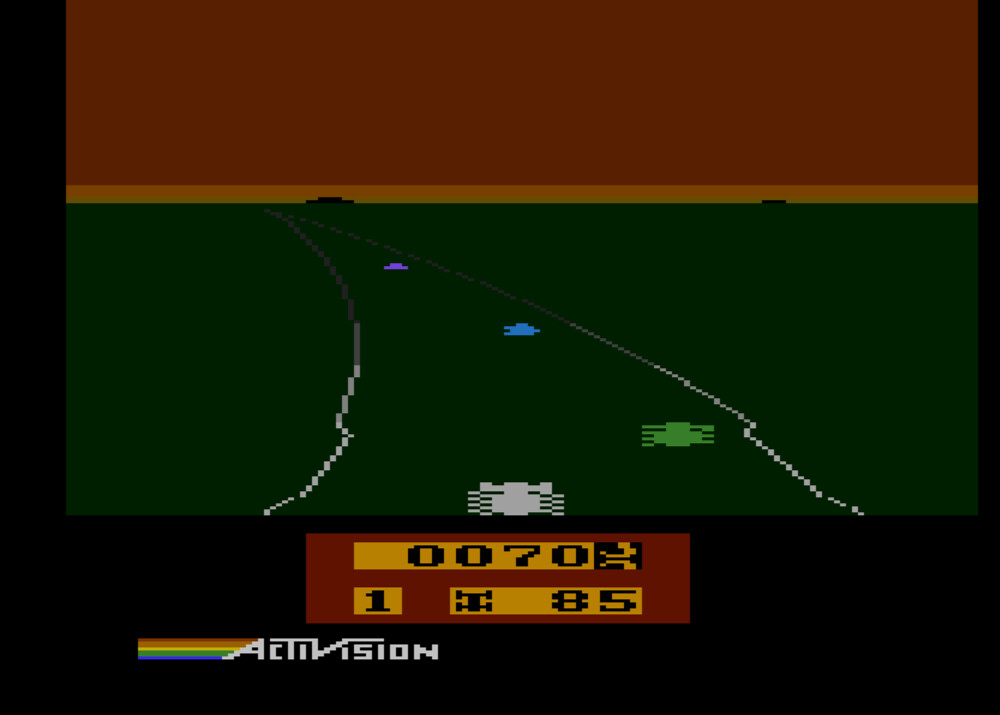This screenshot showcases a classic, pixelated video game that appears to be from the early days of gaming. The majority of the screen is shrouded in black, focusing the viewer's attention on a rectangular area towards the upper section. This rectangle features a brown and green landscape that hints at a rudimentary driving game. A highly pixelated road stretches from the center of the screen towards the upper left, vanishing into the distance.

Scattered across the road are several blocky, spider-like figures in various colors. A white figure, likely representing the player's vehicle, is positioned at the forefront, seemingly navigating the path ahead. To the player's right is a green figure, followed by a blue one further down the road, and a purple figure almost fading into the horizon.

Below this gameplay area, a red rectangular section houses the game’s scoreboard. The scoreboard displays the number "0070," with a "1" underneath it. To the immediate right, another set of numbers reads "85." In the bottom left corner of the screen, the classic Activision logo is prominently displayed, featuring a rainbow arcing towards the first "A" in "Activision."